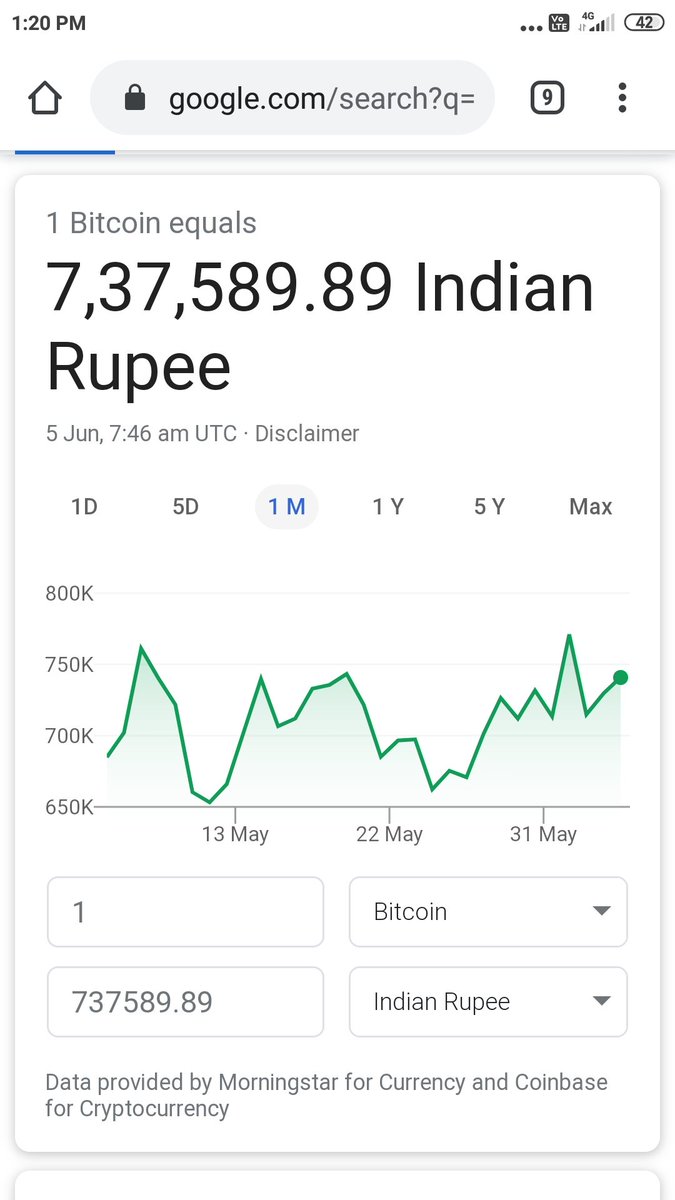In this image, there's a prominently blue outline framing the entire scene. At the top, a small house icon is presented next to the time, reading 1:20 PM. Centrally located is a blue-colored Google search box. Below it, a small black box with the number "9" and three dots is visible. A concise blue line is followed by a longer light blue line, indicating conversion rates.

The conversion rate displayed indicates "1 Bitcoin equals 737,589.89 Indian Rupee." This information is dated the 5th of January at 7:46 AM UTC and is accompanied by a disclaimer.

Beneath this conversion rate, a graphical representation of Bitcoin's value from the 13th of May, through the 22nd of May, to the 31st of May, shows a significant increase towards the end of May. 

Additional blocks beneath the graph provide detailed figures, including a block with "1", a block with "Bitcoin" accompanied by a downward arrow, another block with the value "737,589.89", and one more block with "Indian Rupee" and a downward arrow. It's noted that the data is provided by Morningstar for currency and Coinbase for cryptocurrency.